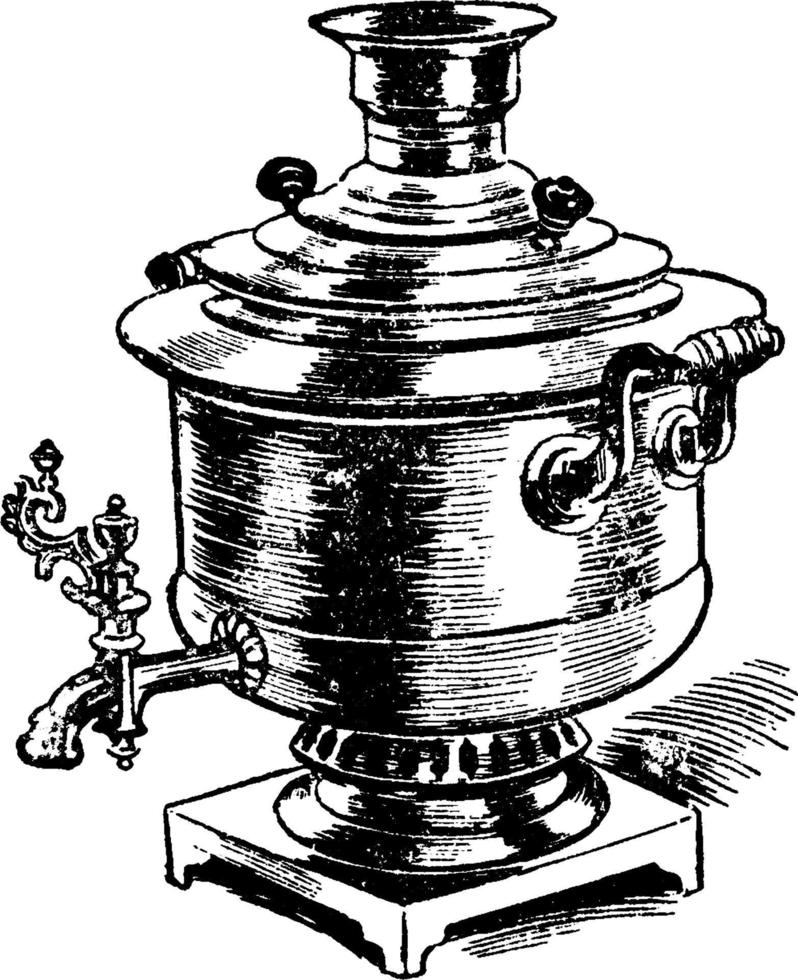This is a detailed black and white ink drawing of a vintage metal kettle, which resembles an old-fashioned water boiler or coffee machine. The kettle features an ornate spout on the left-hand side, with a very intricate, curvy handle that loops around itself. The right-hand side displays visible handles or knobs, and the top narrows into a spigot or valve with a hole in the cap. The machine is set on a small, square stand with feet at each of the four corners. The image background is white with black lines extending upward behind the kettle, adding to the hand-drawn aesthetic. Water lines appear to extend from the back right of the contraption.